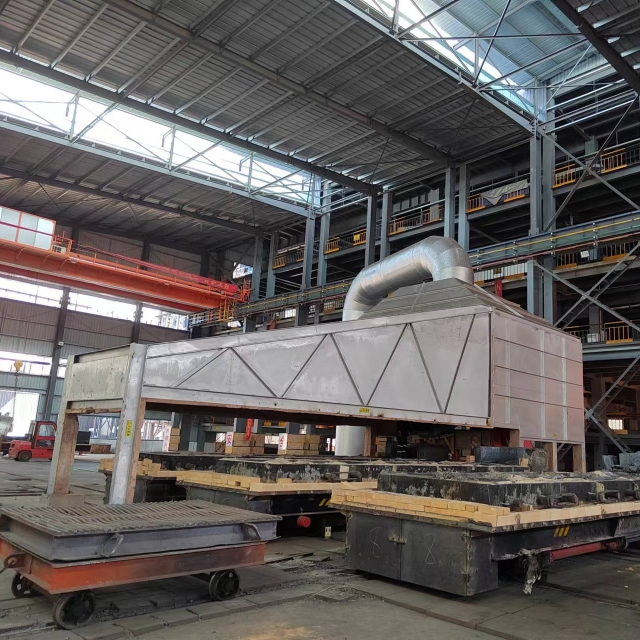The photograph captures the interior of a vast industrial warehouse. Dominating the scene is a humongous piece of machinery, likely a ferroalloy silico manganese furnace, equipped with extensive piping and mounted on dollies resembling railroad flat cars, suggesting it can be moved around. Above the furnace, there are complex exhaust systems, including large metal hoods and a substantial silver pipe extending from the machinery into the ground. Flanking the furnace are three tables with yellow tops, possibly for holding plants or items encased in black, and to the left, a wagon is positioned nearby. In the distance, the high-ceilinged warehouse features an industrial building ceiling with skylights, beams, metal poles supporting the roof, and large windows. The floor is concrete, and various industrial components, including what appears to be a forklift, are faintly visible, adding to the bustling factory ambiance. Overhead, catwalks and cranes are situated amongst a network of struts and beams, emphasizing the functional and industrious nature of the space.